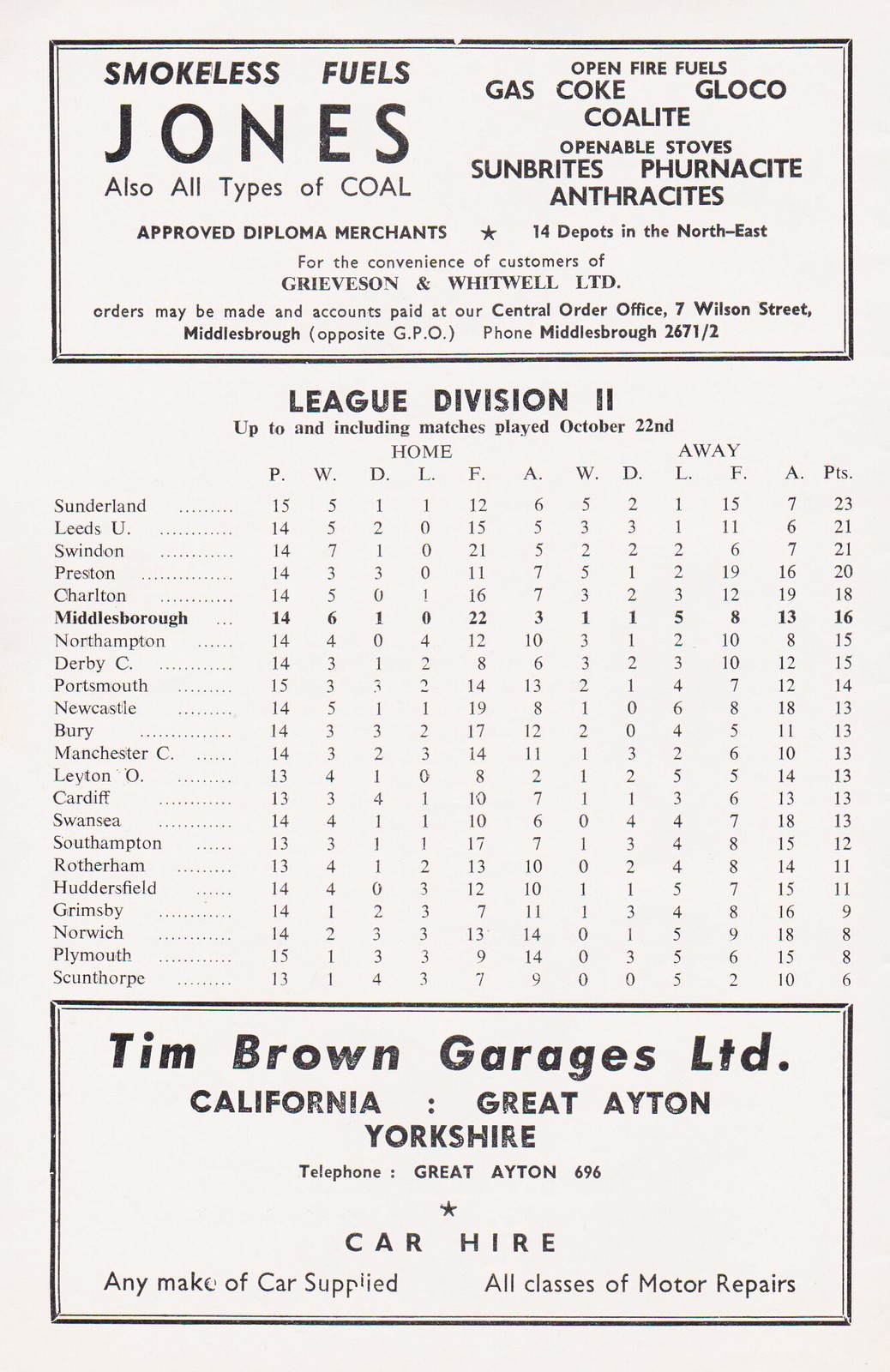The image is a vintage scorecard for League Division II, detailing statistics up to and including matches played on October 22nd. The page is divided into three sections. At the top, within a black rectangular border, is an advertisement for smokeless fuels by Jones, detailing diverse coal types and open fire fuels, including gas, coke, gloco, coalite, and others. It also lists depot information for Grieveson and Whitewell Ltd., providing a central order office at 7 Wilson Street, Middlesbrough, opposite GPO, with the phone number Middlesbrough 62671-2.

The central section of the image meticulously lists the home and away statistics for various sports teams in the league, including Sunderland, Leeds, Swindon, Preston, Charlton, Middlesbrough, Northampton, Derby C, Portsmouth, Newcastle, Bury, Manchester C, Leighton O, Cardiff, Swansea, Southampton, Rotherham, Huddersfield, Grimsby, Norwich, Plymouth, and Scunthorpe. The table includes columns labeled P, W, D, L, F, A for home and away metrics, with total accumulated points on the far right. 

At the bottom, another advertisement for Tim Brown Garages Ltd., located in California, Great Ayton, Yorkshire, features services such as car hire for any make, and all classes of motor repairs. Their contact number is Great Ayton 696.